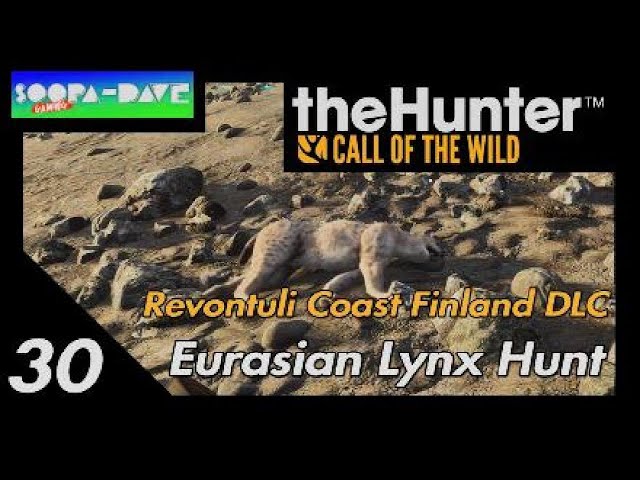The image appears to be a computer-generated scene, possibly from a video game. Set against a black background, the central focus is a dead lynx lying on its side amidst a landscape of tan, brown, and gray rocks and grass. The lynx has its mouth open, giving the appearance of either being injured or deceased. In the upper left corner, there is a blue, green, and white logo for "Supa Dave," while the upper right corner features the logo for "The Hunter: Call of the Wild" in white and yellow font. Overlaid on the lower part of the image is text reading "30 Revontuli Coast Finland DLC Eurasian Lynx Hunt," also in yellow and white font. The image appears to be an advertisement for a hunting game.